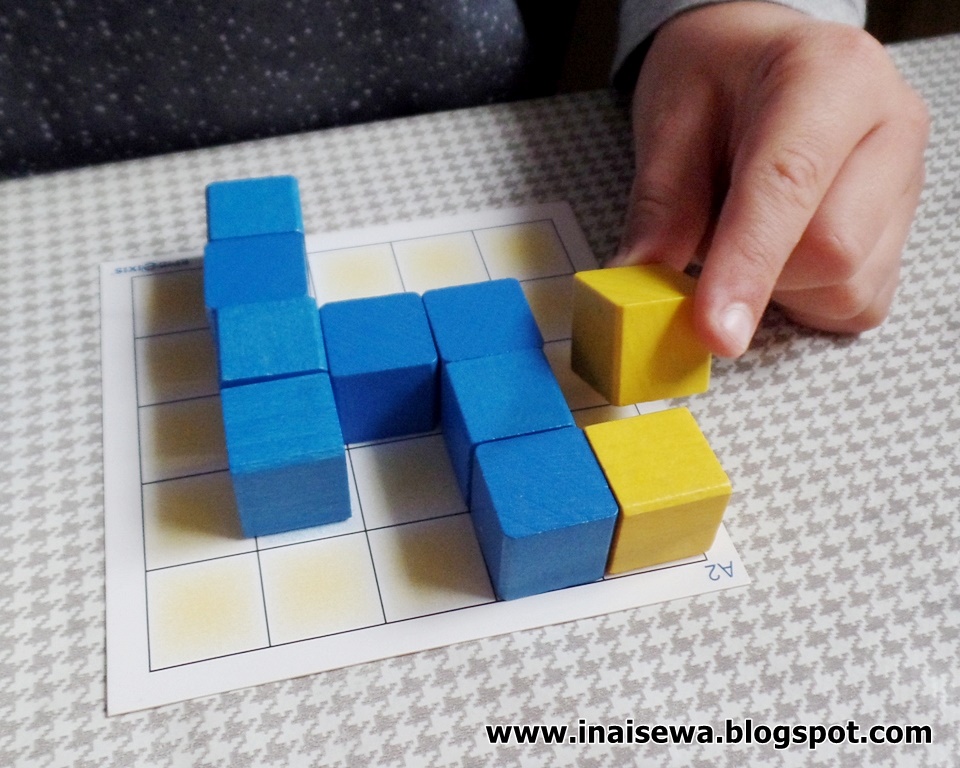In this detailed image, we see a white Caucasian individual holding a vibrant yellow cube in their hand. The individual is dressed in a light grey shirt, which contrasts with the dark, black, speckled background behind them. At the very bottom of the image, in bold black font, the URL "www.inaisewa.blogspot.com" is prominently displayed.

The table in front of the person features a unique, greyish, almost squirrelly pattern distributed across a white surface. On the table lies a white sheet of paper, labelled "A2" at the top. The paper also contains some black font text in the top left corner, though the specifics of the text are unclear.

Adjacent to the white sheet of paper, there are two yellow squares, positioned to the left of a black square-outlined board. The board itself is arranged with three blue cubes aligned vertically, followed by another three blue cubes horizontally, and then four more blue cubes descending vertically. The empty spaces on the board showcase a combination of light yellow and white hues, adding a dynamic visual element to the composition.